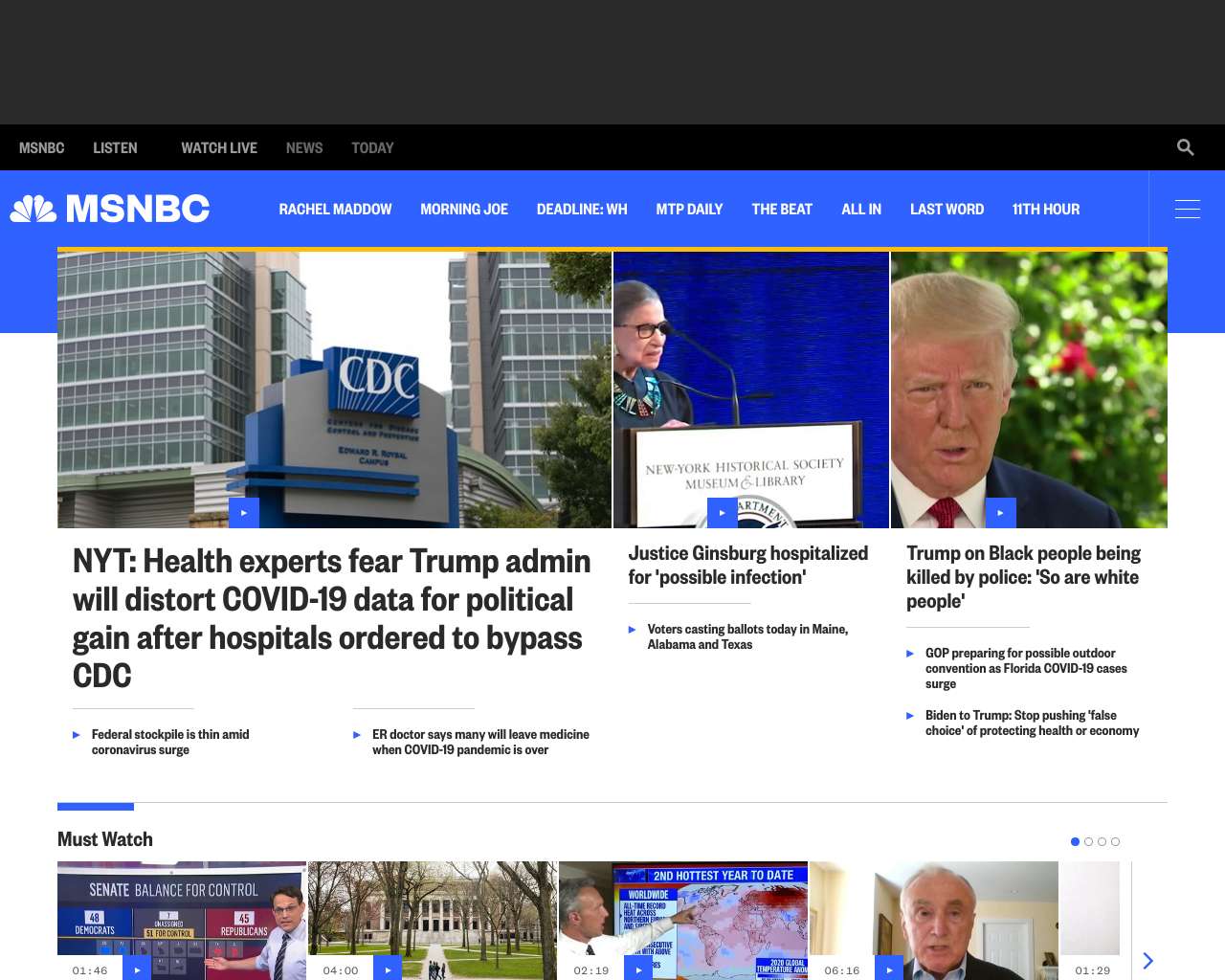The website page from MSNBC features a prominently black top banner, clearly indicating its affiliation with MSNBC. The banner includes options such as "Listen," "Watch Live," and links to the latest news, along with a search bar.

Beneath the banner, the background shifts to a bright blue, featuring the MSNBC logo along with program titles like "Rachel Maddow," "Morning Joe," "Deadline WH," "MTP Daily," "The Beat," "All In," "Last Word," and "WTH Hour." 

Below these listings, various news stories are presented:

1. The first story shows a large image of the CDC headquarters, with two buildings and a blue sign with white lettering reading "CDC" in the middle. The headline reads: "NYT: Health experts fear Trump administration will distort COVID-19 data for political gain after hospitals ordered to bypass CDC." No publication date is provided.

2. Another story headline reads: "Federal stockpile is thin amid coronavirus surge," featuring an ER doctor who claims many will leave medicine when the COVID-19 pandemic is over.

3. In the center, there's an announcement that "Justice Ginsburg hospitalized for possible infection," accompanied by her photograph.

4. A headline states "Trump on black people being killed by police: So are white people," illustrated with an image of Donald Trump.

5. Another article highlights that the "GOP is preparing for a possible outdoor convention in Florida as COVID-19 cases surge."

6. Joe Biden is also featured with a quote directed at Trump: "Stop pushing false choice of protecting health or economy."

Additionally, there is a "Must Watch" section displaying large images:
- The Senate balance for control, featuring MSNBC's election analyst Steve Kornacki.
- A White House image.
- A map indicating weather trends, labeled "Second Northeast Year to Date."
- A photograph of a reporter delivering news.

The page is rich with visual elements and offers an assortment of current news stories, making it a comprehensive source of information.